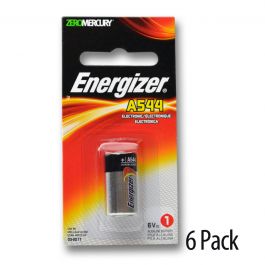The image prominently features a large photo of an Energizer battery packaged for retail. The top section of the package is shaded green with a soft blur, displaying the word "mercury" in white lettering. A small hole at the top of the package suggests that it is designed to be hung on a store rack.

The brand name "Energizer" stands out in bold white letters, with a trademark symbol positioned immediately to the right of the last letter 'R'. The package design incorporates a blend of black, orange, yellow, and a grayish color scheme, typical of Energizer branding. The displayed battery itself is characterized by a black top and a gray bottom, featuring the Energizer logo and name clearly printed on it.

On both sides of the packaging, there is additional text related to marketing and product information; however, it appears blurred and unreadable. Lastly, a small label to the right of the package, not situated on the package itself, indicates that it contains a six-pack of batteries.